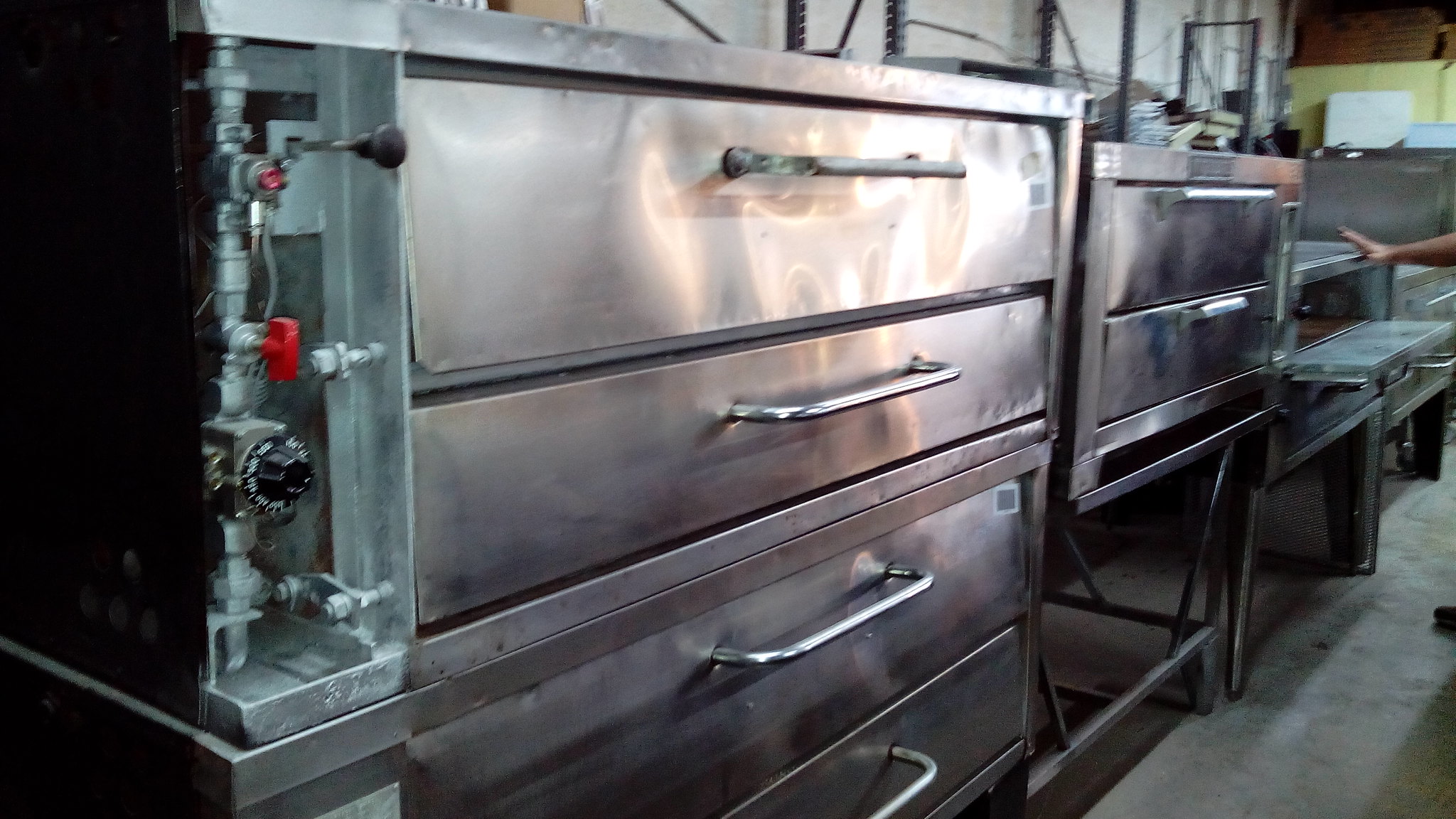The image depicts a bustling industrial kitchen area dominated by sleek, dull silver steel equipment. Central to the photo is an arrangement of wide metal drawers resembling file cabinets, likely used for culinary purposes. On the far right, an open industrial oven is partially visible, with a person's hand resting on it, suggesting ongoing activity. This oven, referenced as potentially being for pizza or other baked goods, hints at the scene being part of a bakery or a similar large-scale kitchen. To the left, various gadgets and dials, possibly for gas controls, are visible alongside a tangle of wiring. The floor is plain, possibly cement, reinforcing the utilitarian feel of the industrial setting. The overall aesthetic is one of functional simplicity, with no text or writing to distract from the focus on the work area.